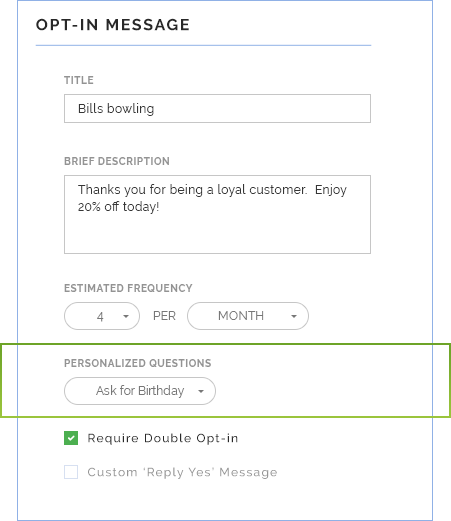Caption: 

The image showcases a webpage under the category "Websites," featuring a user interface for managing opt-in messages. At the top, in bold black text, it reads "Opt-in Message" with a horizontal blue line underneath. Below, there are various labeled sections:

- **Title:** "Bills Bowling" written in solid black text.
- **Brief Description:** "Thank you for being a loyal customer, enjoy 20% off today," displayed in gray text.

The estimated frequency of the messages is set to "four per month" with interactive drop-down menus for both "four" and "month" allowing user customization.

Additionally, there are sections for personalized questions where "Ask for a birthday" is highlighted with a green box around it.

Further down, the interface includes:

- A bolded option titled "Require Double Opt-in," accompanied by a green box with a white checkmark.
- An unchecked blank box labeled "Custom reply yes message."

The text for "Opt-in Message" and "Require Double Opt-in" is bolded, while "Title," "Brief Description," "Estimated Frequency," and "Personalization Questions" are in gray letters, making the key elements stand out prominently against the neutral background.